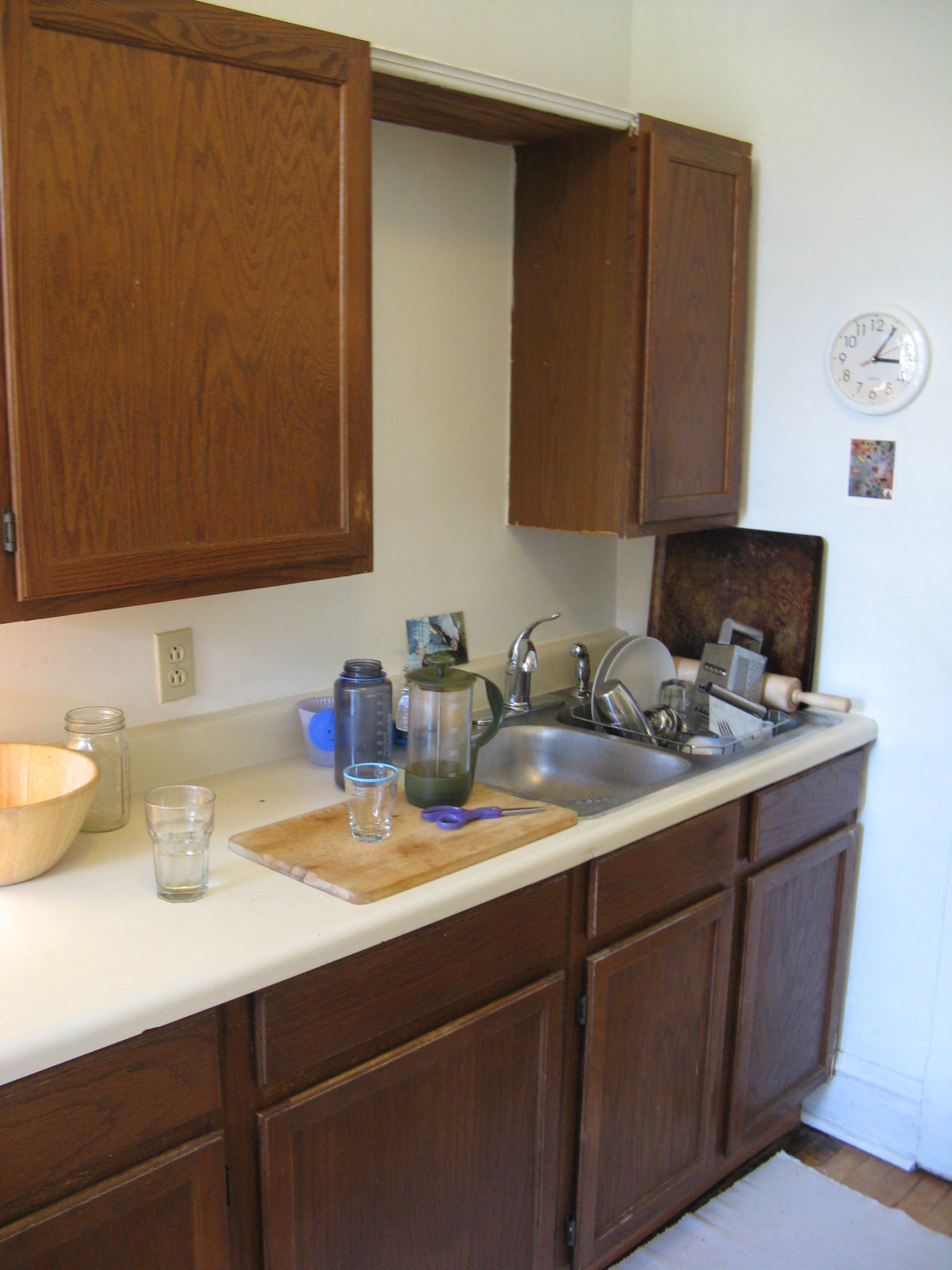This photograph captures a well-used, cozy kitchen space with a focus on the double-sectioned sink situated at the center. The sink itself is divided into two basins by a central faucet. The right basin contains a drying rack brimming with various kitchen utensils and items, including a cheese grater, a stainless steel martini shaker, a few glasses, and bowls. A rolling pin and a cutting board rest neatly to the right of the sink. On the left side, a wooden cutting board lies on the white countertop, accompanied by a pair of scissors, a plastic pitcher, and a glass.

In the background, the pristine white countertop contrasts with the warm brown cabinetry. A white wall clock, positioned to the right, adds a touch of classic charm to the scene. The overall ambience of the kitchen is a harmonious blend of functionality and homey comfort.